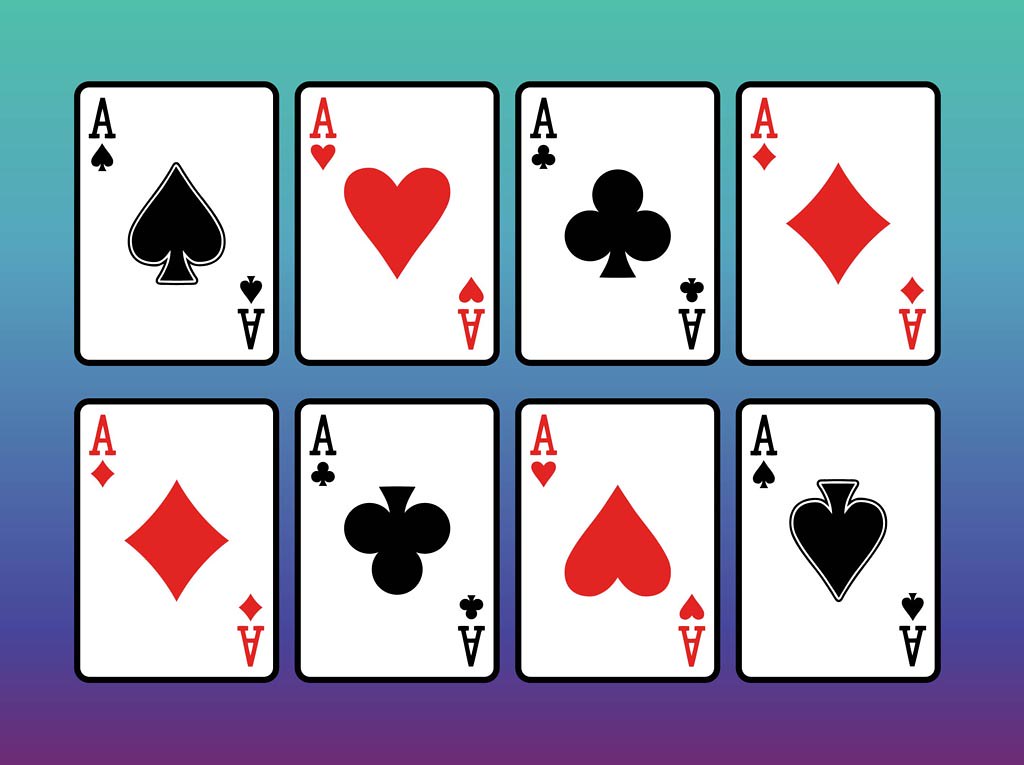The image showcases a computer-generated gradient background that transitions from a matte turquoise green at the top to various hues as it moves downward: first becoming more blue, then blue-green, followed by blue, and eventually blending into purple and light purple at the bottom, resembling a cascading wave of color.

In the foreground, eight computer-generated playing cards are displayed, organized in two rows of four. The top row features the aces of Spades, Hearts, Clubs, and Diamonds arranged from left to right in their upright positions. The bottom row mirrors the same sequence—Ace of Spades, Ace of Hearts, Ace of Clubs, and Ace of Diamonds—but these cards are positioned upside down.

This richly colored, digitally crafted artwork provides an intriguing contrast between the vibrant gradient background and the classic design of the playing cards, emphasizing the symmetry and uniformity intrinsic to this computer-generated scene.